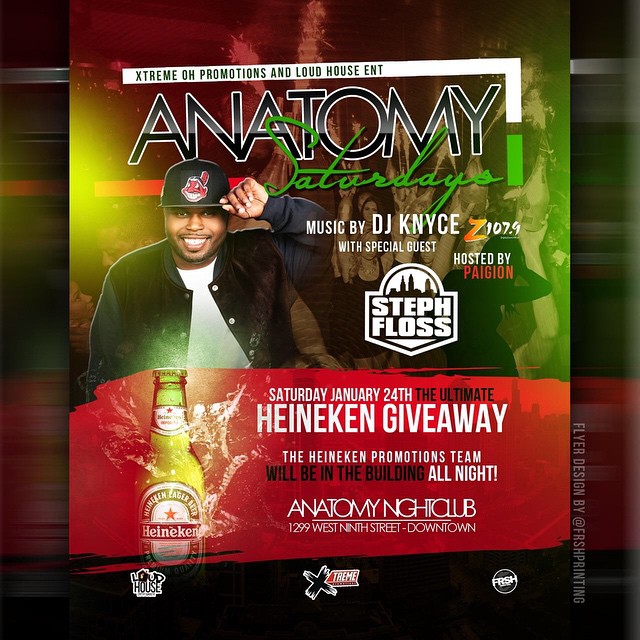This advertisement, dominated by red and black hues, promotes an event called "Anatomy Saturdays," organized by Extreme OH Promotions and Liquid House Entertainment. The event features music by DJ KNYCE and special guest Steph Floss, and is hosted by Pagan with Z107.9. The central figure of the poster is a young African American man, likely DJ KNYCE, wearing a black Cleveland Indians baseball cap and a black jacket over a white t-shirt. He is smiling, showcasing his dark brown eyes and goatee. The event, scheduled for Saturday, January 24th, highlights a Heineken giveaway with the Heineken Promotions team present all night. The poster, which also shows a prominently placed bottle of Heineken beer, mentions the venue as Anatomy Nightclub, located at 1299 West 9th Street, downtown.